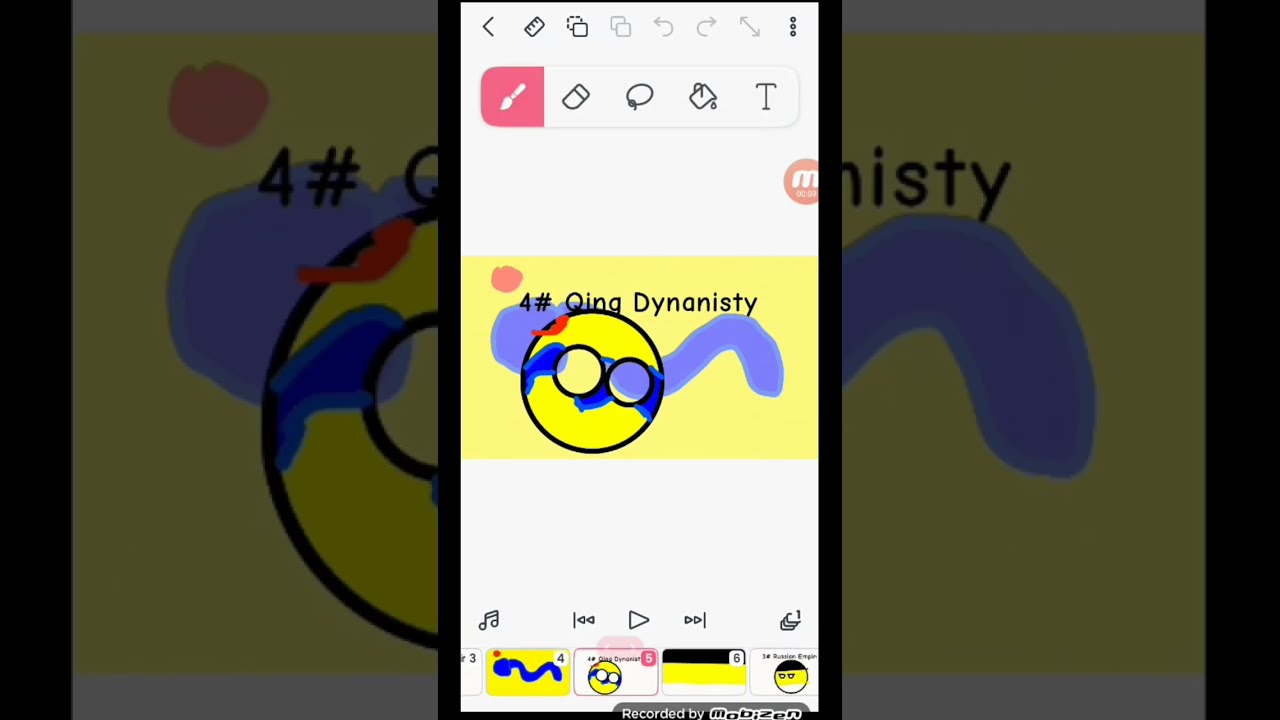This image depicts a close-up view of a cell phone screen displaying a drawing application. The phone's black outline is partially cut off at the top and bottom, revealing a mostly white background. The user interface at the top features various icons including a backspace button, a ruler, and navigation arrows. Below this is a tool selection with a highlighted pink paintbrush, an eraser, a ring-like circle, a paint can, and a text ('T') option. 

In the center of the screen, there's a distinctive yellow horizontal stripe with a darker yellow circle outlined in black, resembling a face with black-rimmed glasses, alongside a blue squiggly line. Above this graphic, in black text, it reads "4 #Queen Dynasty." At the bottom of the screen, playback controls are visible, including a play button, fast forward, and rewind, along with a musical note and other symbols. 

The cell phone itself is placed against an enlarged, grayed-out version of its own screen, making the central yellow stripe and graphic appear larger in the background, extending to the left and right of the phone. The overlay effect creates a repeated, magnified look of the key elements on the screen. The caption "recorded by Moe Dizit" is noted in black and white at the bottom on a gray background.